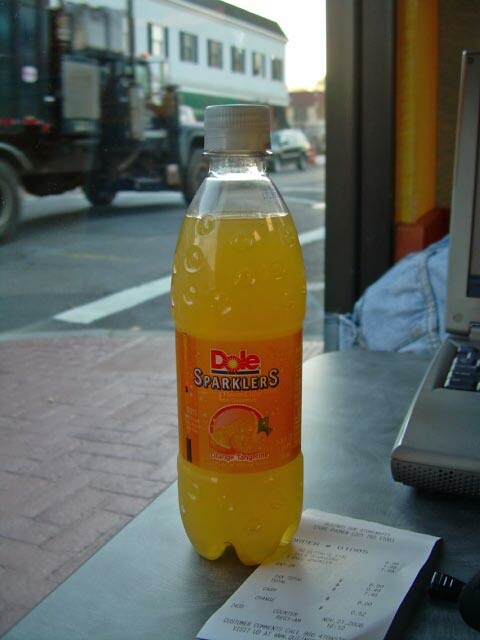This photograph offers a glimpse through a window from inside a building, capturing a scene that stretches out to a road in the distance. The road is dotted with vehicles that evoke a sense of nostalgia, resembling vintage farming trucks or old-style automobiles. Anchoring the foreground is a full bottle of an orange-colored beverage, prominently bearing the label "Dull Sparklers" alongside an image of an orange, and the text "Orange Tangerine." Beneath the bottle lies a receipt adorned with black text. To the side of the frame, the edge of an old-fashioned laptop computer is discernible, adding to the scene’s quaint atmosphere.